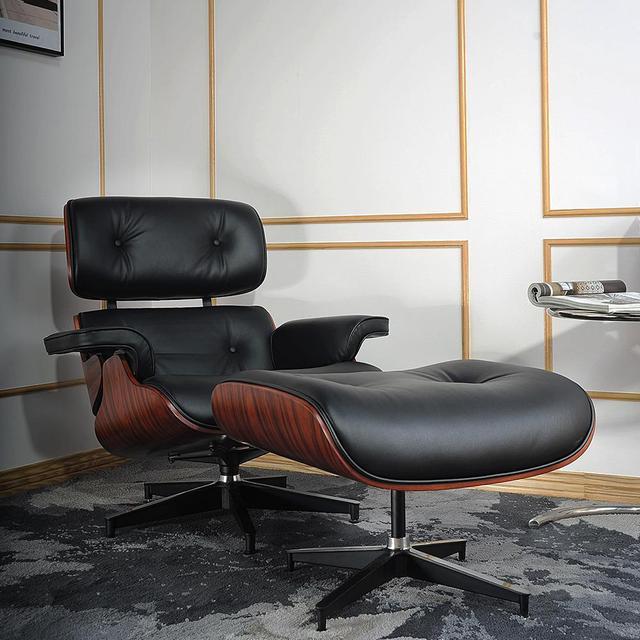The image showcases a meticulously arranged corner of a room. The walls are pristine white, each adorned with rectangular gold outlines that add a touch of elegance and symmetry. The corner of the room is positioned on the left-hand side of the frame, partially revealing a black-framed photograph that contributes an artistic element to the setting. 

Dominating the scene is a sleek, black leather chair, featuring a smooth mahogany wooden base. The chair is relatively short and has arms that gracefully fold upward and outward, made of the same luxurious black leather material. It rests on a sturdy base consisting of five prongs, each equipped with small wheels for easy mobility.

Adjacent to the chair is a footstool, slightly elevated and mirroring the chair’s design with a mahogany underside and black leather upholstery. A hint of modernity is added by a silver table beside the chair. Only the curved, metallic foot of the table is fully visible, hinting at its contemporary design. Atop the table rests a book or magazine, casually folded over on one side, suggesting a momentarily paused reading session.